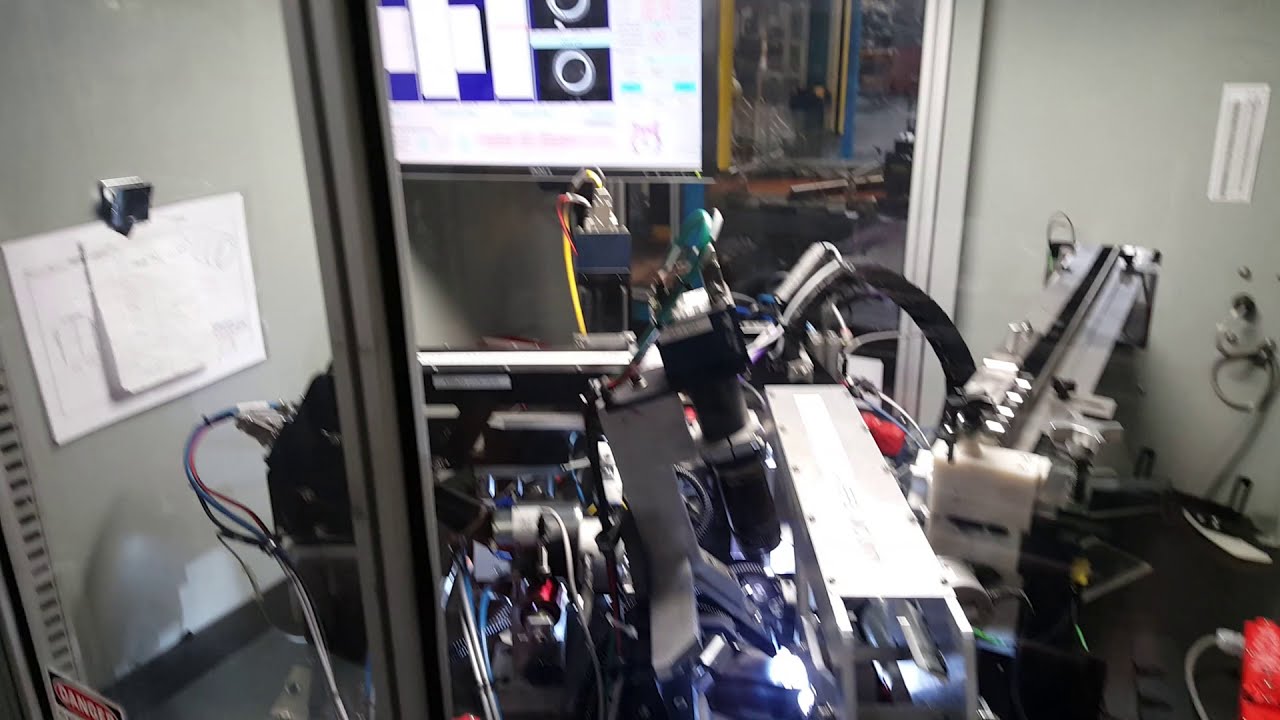The photograph features an office-like room densely packed with various electronic machinery and intricate mechanical components. The machinery, primarily in shades of silver, black, and white, is interconnected with numerous wires and tubes, suggesting a complex, potentially hazardous setup as indicated by the red, white, and black "Danger" sign visible in the bottom left corner. The walls of the room are light gray, with the left wall adorned with two sheets of paper clipped together by a large metal clip. In the background, a doorway leads into another cluttered room filled with additional objects. Adjacent to this doorway, a monitor is mounted on the right-hand wall, displaying an array of black, blue, white, and turquoise squares and rectangles. The right wall also features another piece of white paper, taped onto it. The overall scene is somewhat chaotic and visually intricate, with many details pointing towards a high-tech, possibly industrial environment.